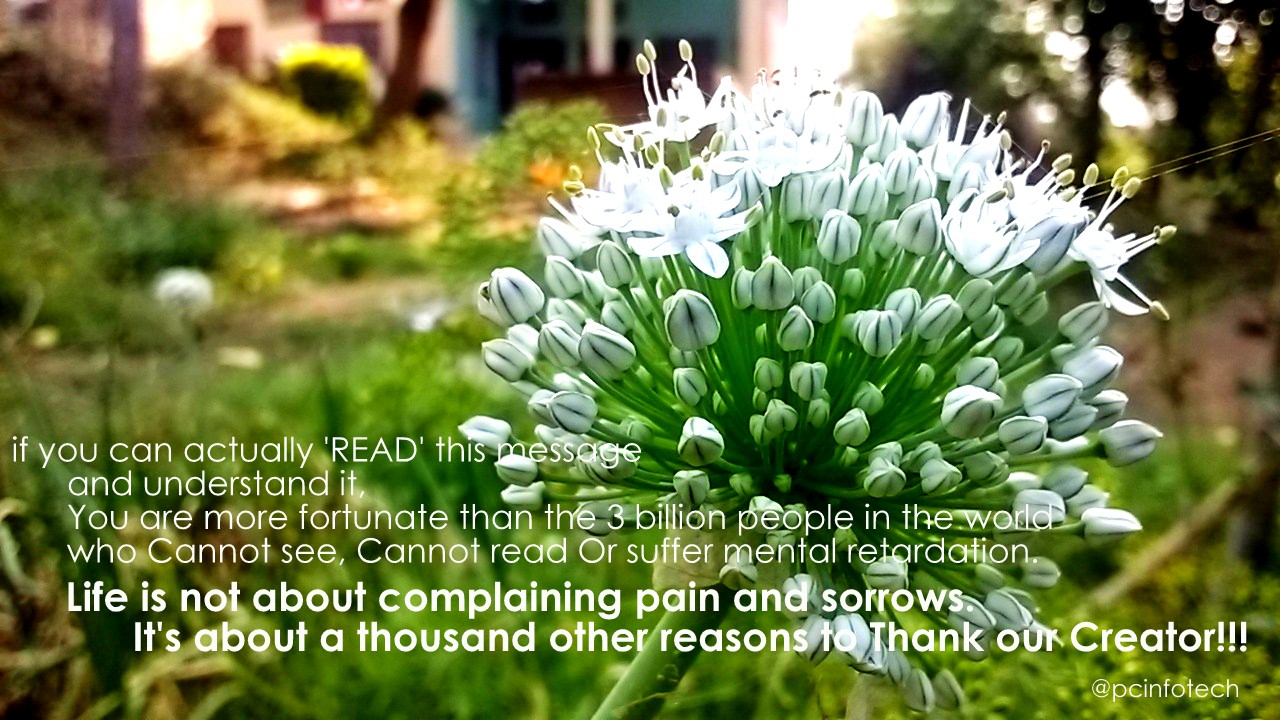A close-up photograph features a vibrant green plant in sharp focus, set against a softly blurred background of additional greenery. Prominently displayed in white text are the words, "If you can actually READ this message and understand it, you are more fortunate than the three billion people in the world who cannot see, cannot read, or suffer mental retardation. Life is not about complaining, pain, and sorrows. It's about a thousand other reasons to thank our Creator." The word "READ" is in all caps, emphasizing the message's significance. The words "thank" and "Creator" are notably capitalized for emphasis. In the bottom right corner, in smaller, lowercase letters, the source "at PC InfoTech" is credited. The image's shallow depth of field accentuates the clear, bright green plant in the foreground, creating a striking visual contrast with the softly blurred green background, ensuring the focus remains on the thoughtful and motivational message.